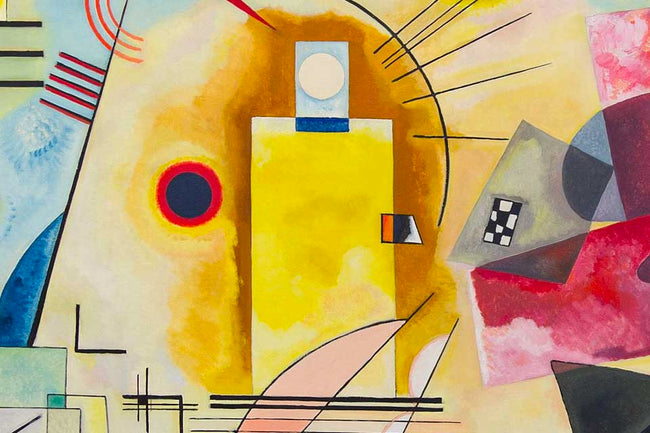This vibrant and intricate abstract watercolor painting on a rectangular canvas is teeming with a diverse array of shapes and vivid colors. Dominating the composition, a yellow background provides a bright backdrop to a plethora of forms scattered across the canvas. On the right-hand side, a pink triangle and a gray-and-maroon colored circle or oval catch the eye, adjacent to a transparent square with a grayish checkerboard pattern. Just below this, a striking red rectangle and a black triangle sit in the bottom right corner. The canvas also features a noteworthy large shape on the left side, reminiscent of a head outlined in black, with detailed elements such as brown-lined 'hair', an abstract yellow rectangular nose, and eyes of different shapes, with a white dot adorning the forehead. 

Intriguing elements like a checker box on the right and a black dot with a red outline contribute to the complex narrative of the piece. A yellow strip slices across the middle of the work, while various colors such as light blue, orange, red, green, gray, dark purple, and white interplay throughout. Some parts of the image feature black parallel lines near the bottom and red lines crisscrossing the left side. The artwork's layering and overlapping of shapes and colors, as well as the fluid blending of pigments, suggest a harmonious blend of watercolor techniques and marker-defined lines. The overall impression is a captivating mosaic of diverse geometric forms, vibrant hues, and intriguing patterns, making it a striking representation of abstract artistry.